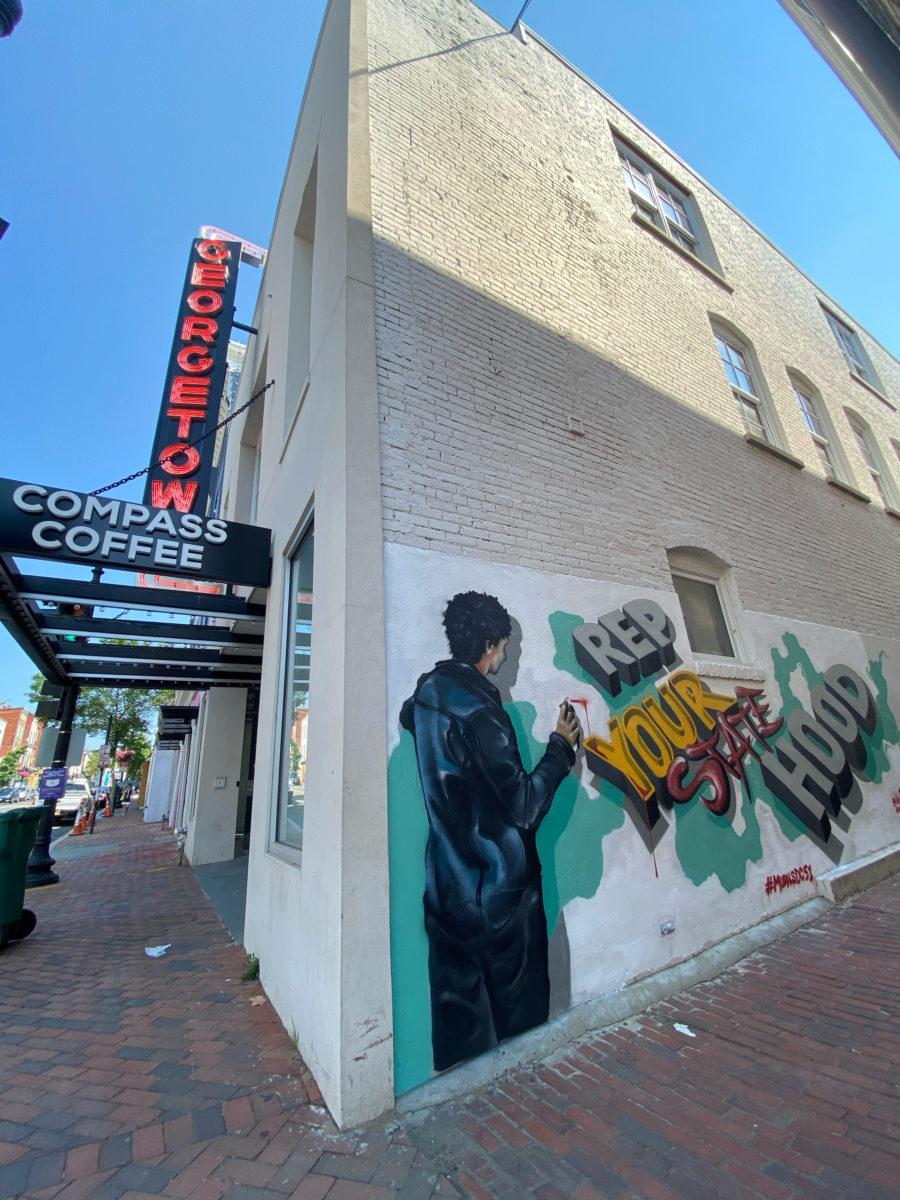This image captures the vibrant corner of an office building set in a downtown area. The building, primarily composed of light-colored brick, prominently features the names "Georgetown" and "Compass Coffee." "Georgetown" is displayed in striking red neon lights against a black background, though the "N" is partially obscured from view. Situated directly beneath, the "Compass Coffee" sign is embossed in clean white lettering. 

Flanking the building is an engaging mural that notably reads "Rep Your Statehood" in a combination of gray and varying colors. This mural is three-dimensional in style, lending it a realistic, protruding look. Central to the mural is the figure of a man, dressed in black overalls, seemingly in the act of spray-painting the wall, creating a captivating illusion. A hashtag, rendered in red, punctuates the artwork towards the bottom.

The immediate surroundings include a well-maintained brick sidewalk, marked with safety cones and a trash can, contributing to its urban charm. The scene is devoid of pedestrians but is enriched with the presence of nearby trees, cars, and other structures. A clear blue sky forms a vivid backdrop, enhancing the building's aesthetic appeal.